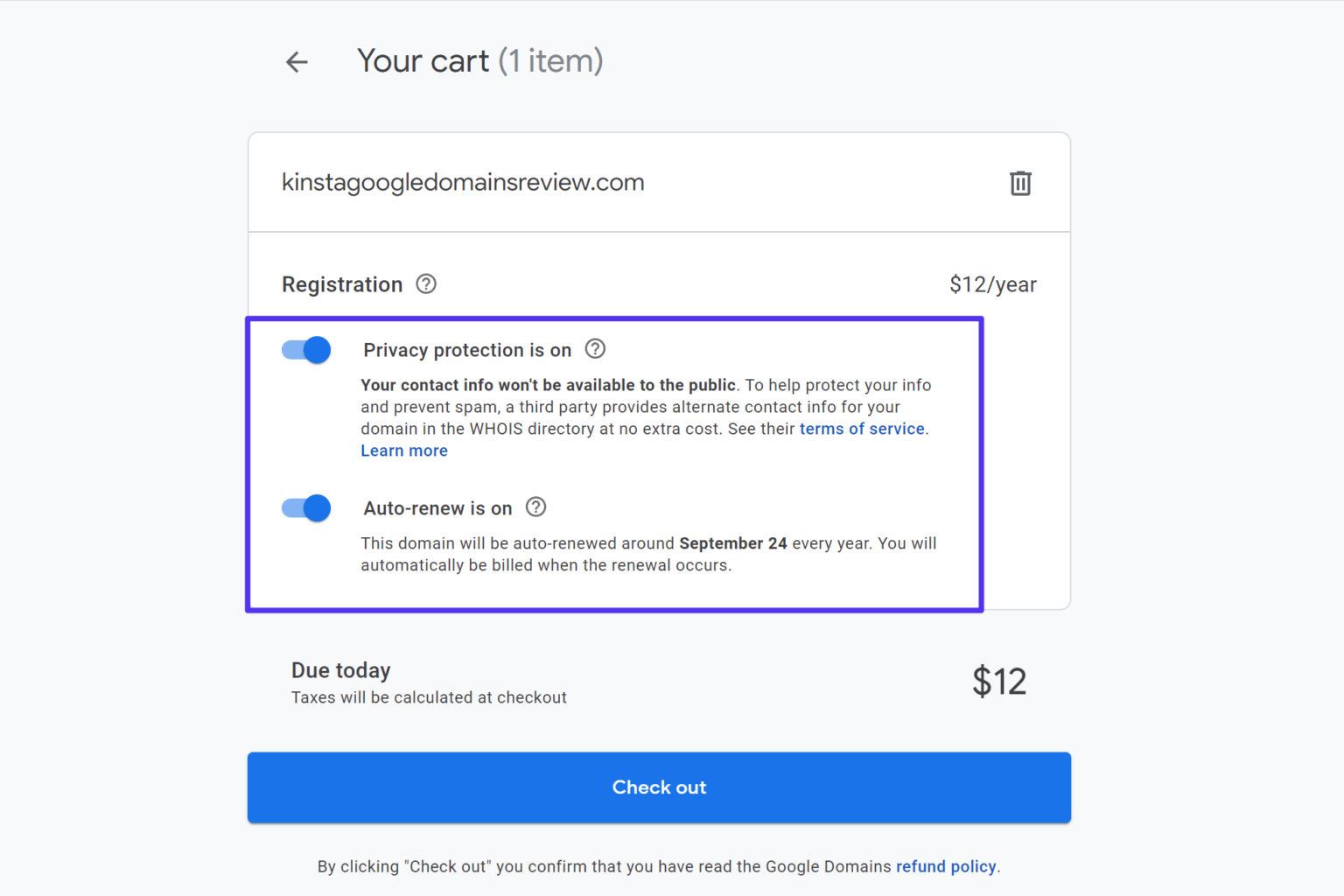The image depicts a detailed interface of a shopping cart on a light gray background. At the top, there is a black arrow pointing to the left, followed by the text "Your cart" in black, and "1 item" in gray parentheses. Directly below, there's a web address: "kinstagoogledomainsreview.com," accompanied by a small trash can icon. 

A horizontal line separates this header from the section below. Under this line, black text reads "Registration," accompanied by a question mark inside a circle. The cost is stated as "$12/year." Next, there is a blue-outlined box containing two toggles, both turned on.

The first toggle section is titled "Privacy Protection is ON" with a question mark inside a circle. This section elaborates that the user's contact information will not be publicly available to protect privacy and reduce spam. It notes that a third party will provide alternate contact information for the WHOIS directory at no extra cost, with clickable text links "terms of service" and "learn more," both in blue.

The second toggle section is titled "Auto-renew is ON," also followed by a question mark inside a circle. It specifies that the domain will auto-renew around September 24th each year, and the user will be automatically billed upon renewal.

Beneath this, it states "Due today" with a note that taxes will be calculated at checkout, and the amount due is "$12." At the bottom, there is a large blue “Checkout” button, accompanied by a statement underneath: "By clicking Checkout, you confirm that you have read the Google Domains refund policy."